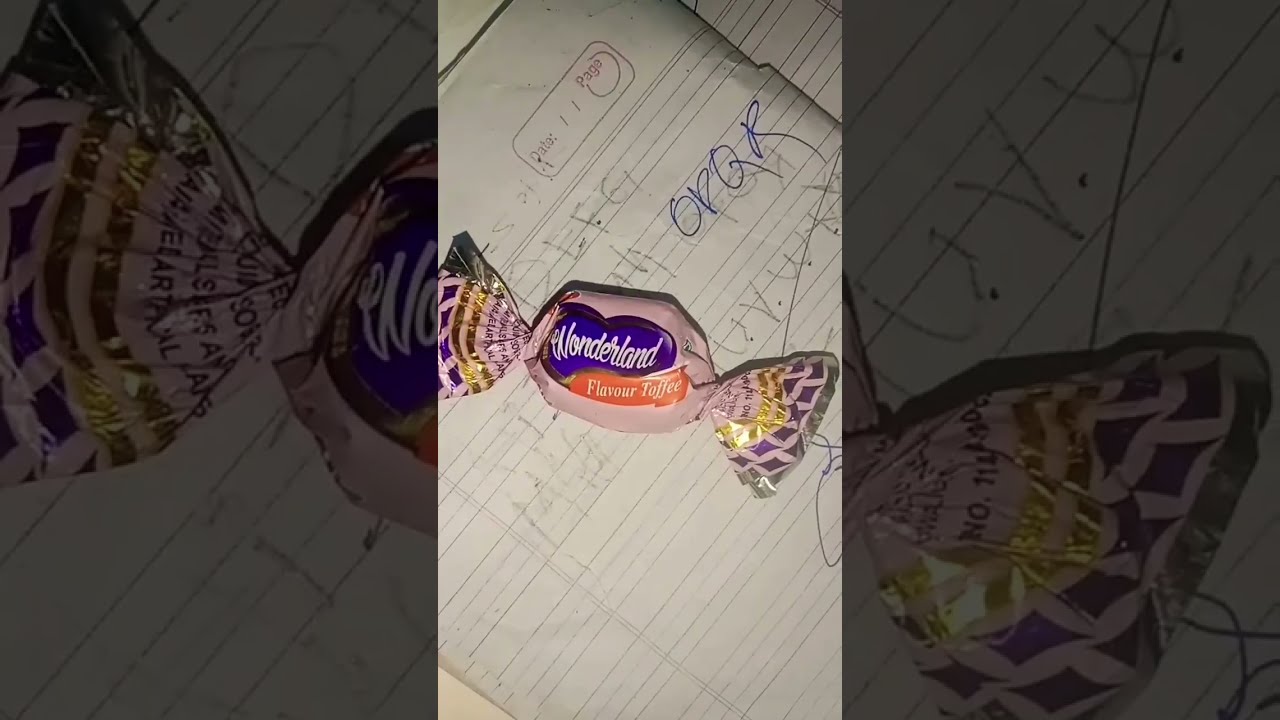The image features a detailed scene centered around a tall, rectangular photograph of a round piece of candy resting on a notebook. The candy, wrapped in a pink plastic wrapper adorned with purple and gold designs, is labeled "Wonderland" on a blue background, with "Flavor Toffee" written below on an orange background. The wrapper is twisted at the sides, creating a bow-like appearance. Flanking the central photograph are wider, darker close-up shots of the same candy. The background notebook, tilted so the lines slope from left to right, contains pencil drawings and blue pen markings, including areas where the pencil has been smeared or erased. The paper, with sections for date and page number, adds to the textured and slightly chaotic backdrop, with slivers of a beige surface peeking from the bottom left and top left corners.